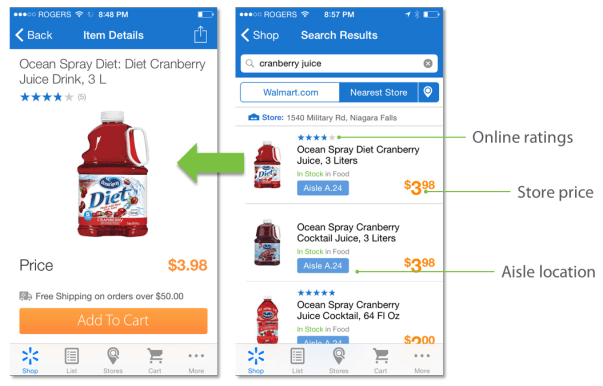This image, likely from the Walmart app, is split into two sections, providing different views of the shopping interface.

**Left Image:**
- The focal point is a product image situated in the middle, displaying a drink with a red liquid, labeled as "Ocean Spray Diet Cranberry Juice Drink 3L." The bottle features a white cap and a red handle.
- Above the product image, the title "Ocean Spray Diet, Diet Cranberry Juice Drink 3L" is prominently displayed.
- Directly below the title, the product rating is shown as 4 out of 5 stars.
- Under the product image, the price is listed as "398" in bold, orange text.
- Further down, a white "Add to cart" button is visible against an orange background.
- At the very bottom left corner, navigation options read "Shop, List, Stores, and Cart."

**Right Image:**
- This section showcases the search results page from the same Walmart app.
- At the top center, "Search results" is displayed.
- Beneath the title, a search box contains the text "cranberry juice" in black.
- Below the search box, there are two tabs: "Walmart.com" on the left and "Nearest store" on the right.
- Three product images are listed beneath these tabs:
  - The first product matches the one from the left image: "Ocean Spray Diet Cranberry Juice Drink 3L" with an arrow pointing to its details.
  - The second product is labeled as "Ocean Spray Cranberry."
  - The third product is identified as "Ocean Spray Cranberry Juice Cocktail."

This comprehensive description provides detailed information about the layout and content of the Walmart app's product listing and search result features.